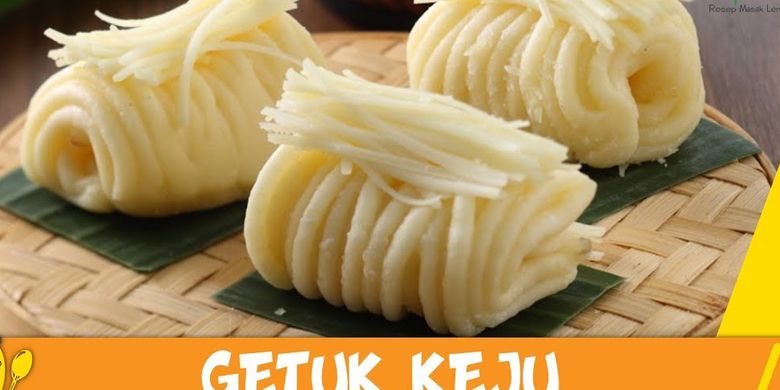The image depicts a beautifully arranged platter of food set atop a woven beige basket, possibly serving as the lid. The food consists of three distinct bundles of curled noodles, resembling sushi noodles or spaghetti, each meticulously placed on small, square green mats that appear to be cut leaves. These mats are dark green and perfectly square, deviating from typical leaf shapes. Each noodle bundle is topped with thin, shredded cheese, which is white and arranged perpendicular to the direction of the noodles. At the bottom of the image, there is an orange band with white, all-caps text in a cartoony, sans-serif font, which reads "GETUK KEJU."